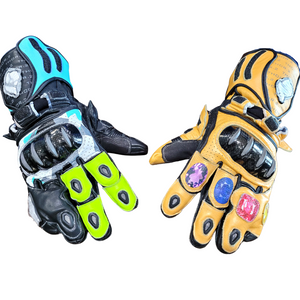In this detailed image, we see a pair of sophisticated motorcycle or biking gloves set against a white background, viewed from the back. The glove on the left, designed for the right hand, is predominantly black with vibrant accents. It features green coloring on the middle and ring fingers, while the rest of the fingers remain black. There's a striking blue and green section near the wrist, and a black strap for fastening. The glove also exhibits blue detailing where the fist would form, complemented by light brown and black stripes extending towards the wrist.

The glove on the right, tailored for the left hand, showcases a primarily light brown or orange hue with intricate black stripes. Its fingers are adorned with an array of colors at the knuckles, including blue, red, and purple, which form circular patterns. The fingertips are distinguished by black tips, and the fist area is marked by a black section. Additionally, there are yellow and black elements on the thumb, and several black lines crisscross near the wrist enhancing its decorative appearance. Both gloves, potentially leather, combine functionality and aesthetics, making them fitting for avid motorcycle racers or extreme sports enthusiasts.